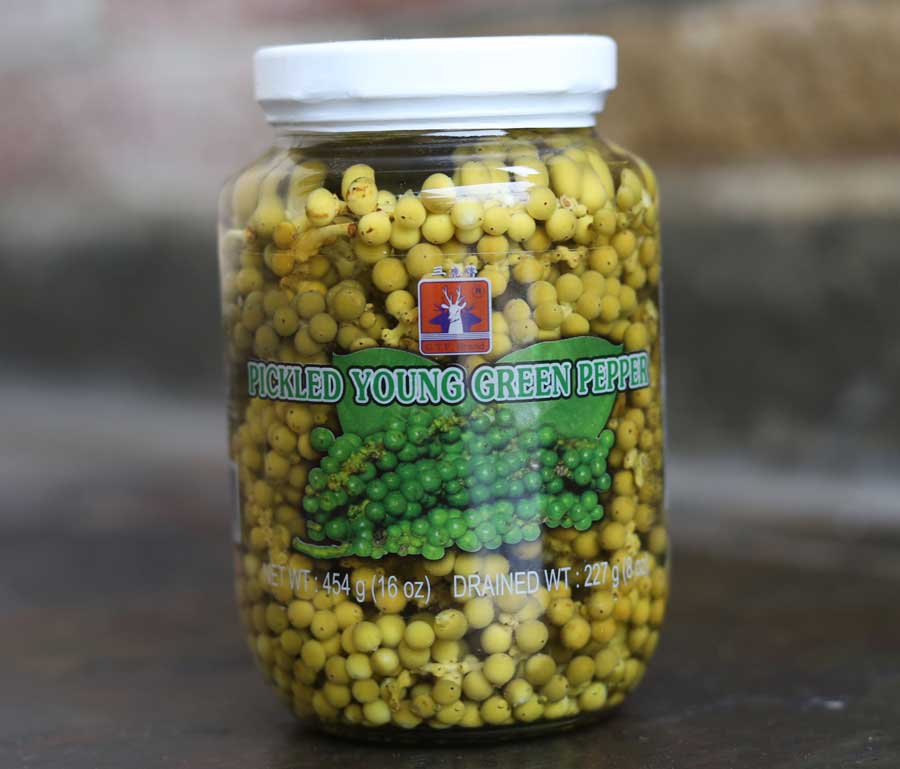This image depicts a clear glass jar with a white lid, containing pickled young green peppercorns. The jar is a standard 16-ounce container, with the contents appearing as small, pea-sized olive green pearls. Featured prominently on the jar's transparent label is an image of a bundle of green peppercorns against green leaves. The label also includes a distinctive logo: a white deer on a red background, framed by a rounded square with a white border. Above the logo, there's text in what seems to be Chinese or Japanese characters. The label provides details about the jar's contents, indicating a net weight of 454 grams (16 ounces) and a drained weight of 227 grams (8 ounces). The photograph shows the jar placed on a table, with the background blurred out, emphasizing the details of the jar itself.